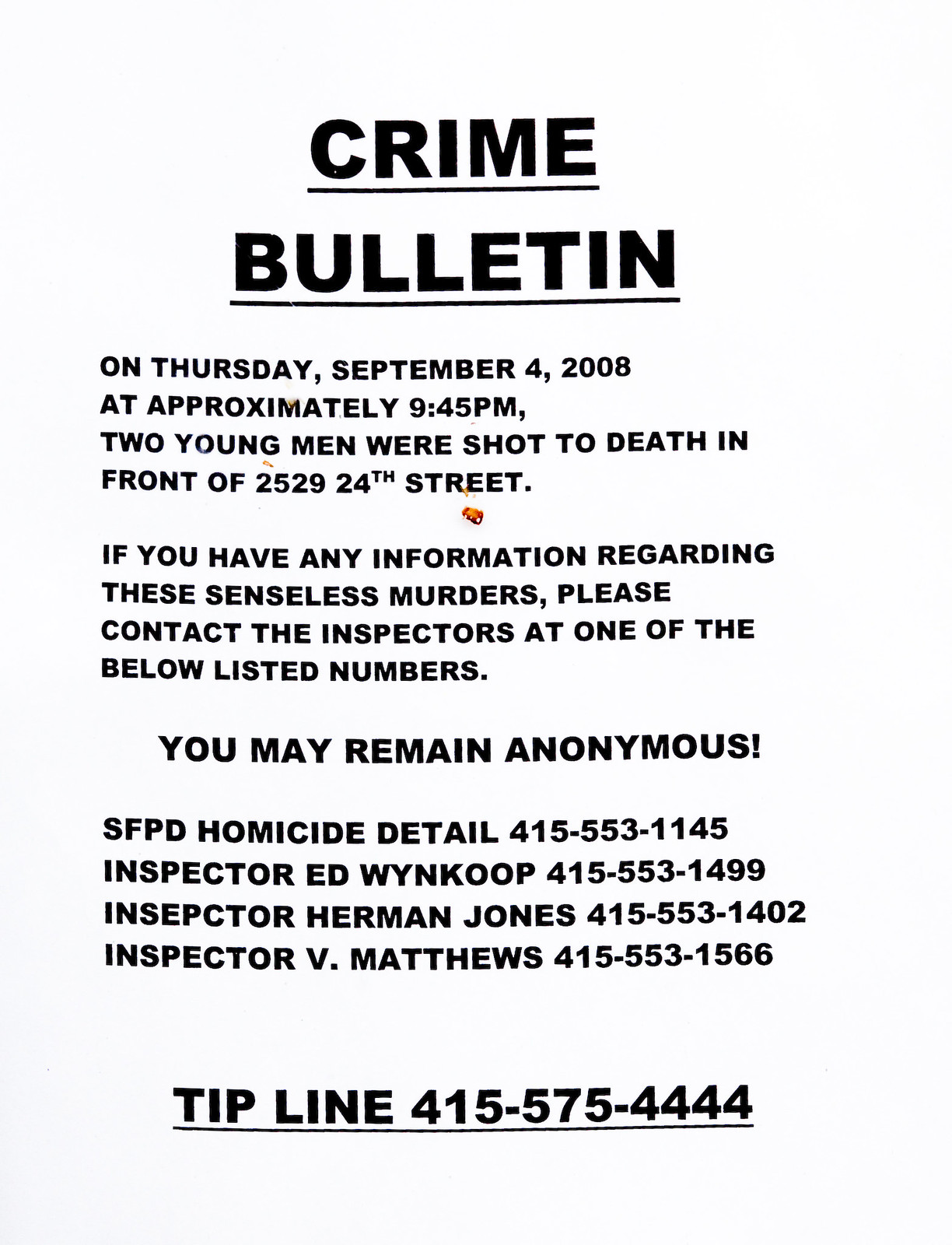A printed out black-and-white crime bulletin centered on a piece of white paper features bold, underlined heading in all capitals "CRIME BULLETIN." Below it, the notice details in black capital letters: "On Thursday, September 4, 2008, at approximately 9:45 p.m., two young men were shot to death in front of 2529 24th Street." The next paragraph urges anyone with information regarding these senseless murders to contact the inspectors at the listed numbers and assures anonymity: "You may remain anonymous." Following this, the bulletin lists the contact details for SFPD Homicide Detail and several inspectors including Inspector Ed Wynkoop at 415-553-1499, Inspector Herman Jones at 415-553-1402, and Inspector V. Matthews at 415-553-1566. At the bottom, in bold, all capital letters, and underlined, it prominently displays: "TIP LINE 415-575-4444." The text is consistently in bold black, emphasizing the gravity and urgency of the message.